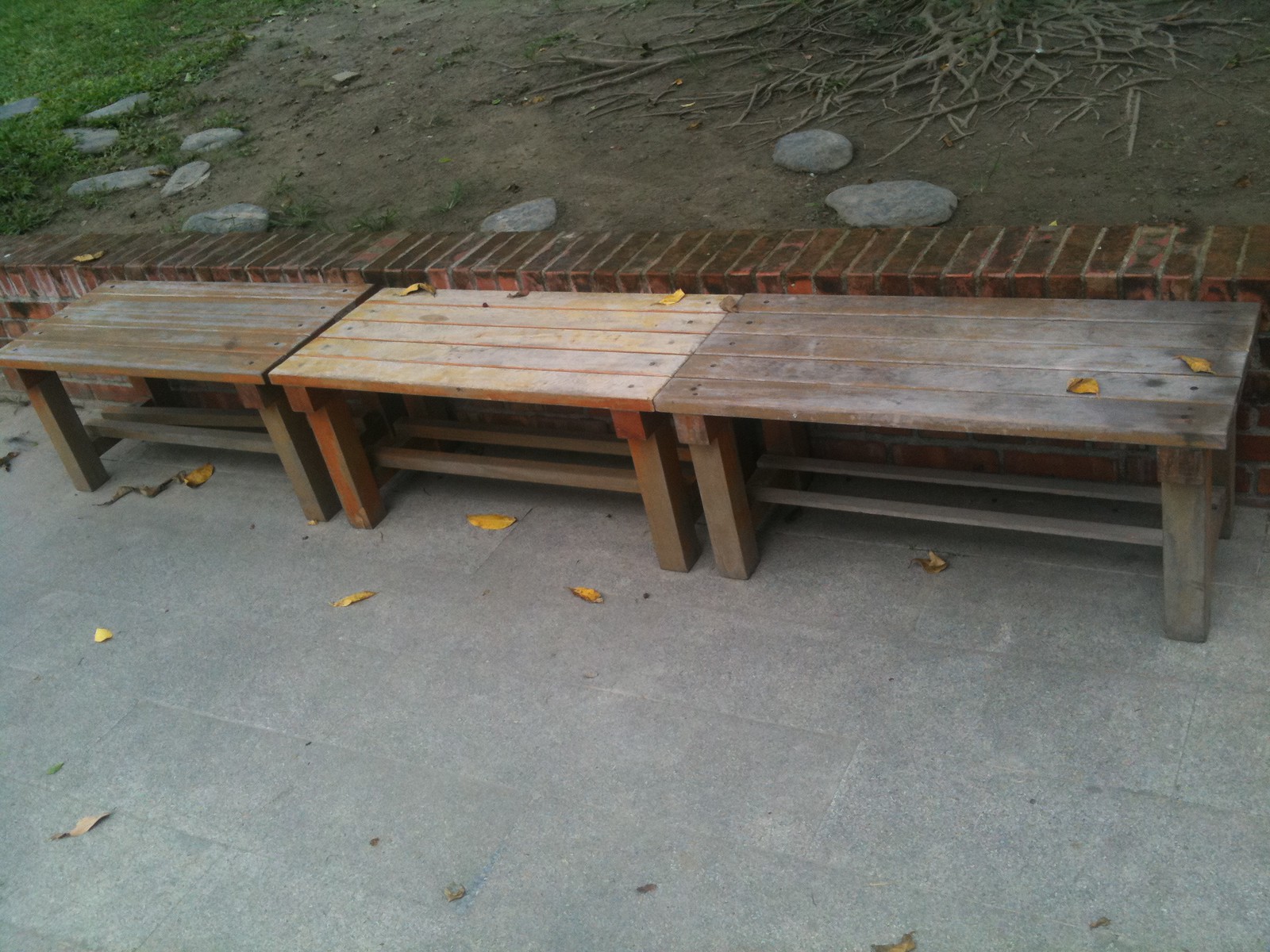This outdoor image captures a slightly wider-than-tall perspective, showcasing three wooden benches arranged horizontally in the center. These benches, positioned diagonally in the shot, rest against a low red brick wall that's about the same height as the benches themselves. The wall is constructed vertically, contrasting the horizontal planks of the benches. The benches vary in color and wear, with the middle bench a lighter, newer wood, while the outer two are medium to dark wood with a weathered look, indicating they have been there for some time.

The benches lack backrests, featuring simple square legs and slatted tops, with some semblance of storage trays underneath. They sit atop a stone walkway made up of large, rectangular gray pavers, speckled with fallen leaves. Beyond the brick wall lies a dirt area crisscrossed with spindly tree roots, large circular stones, and patches of green grass. This backdrop also contains several sticks and gold-colored leaves, enhancing the natural, rustic atmosphere of the scene.